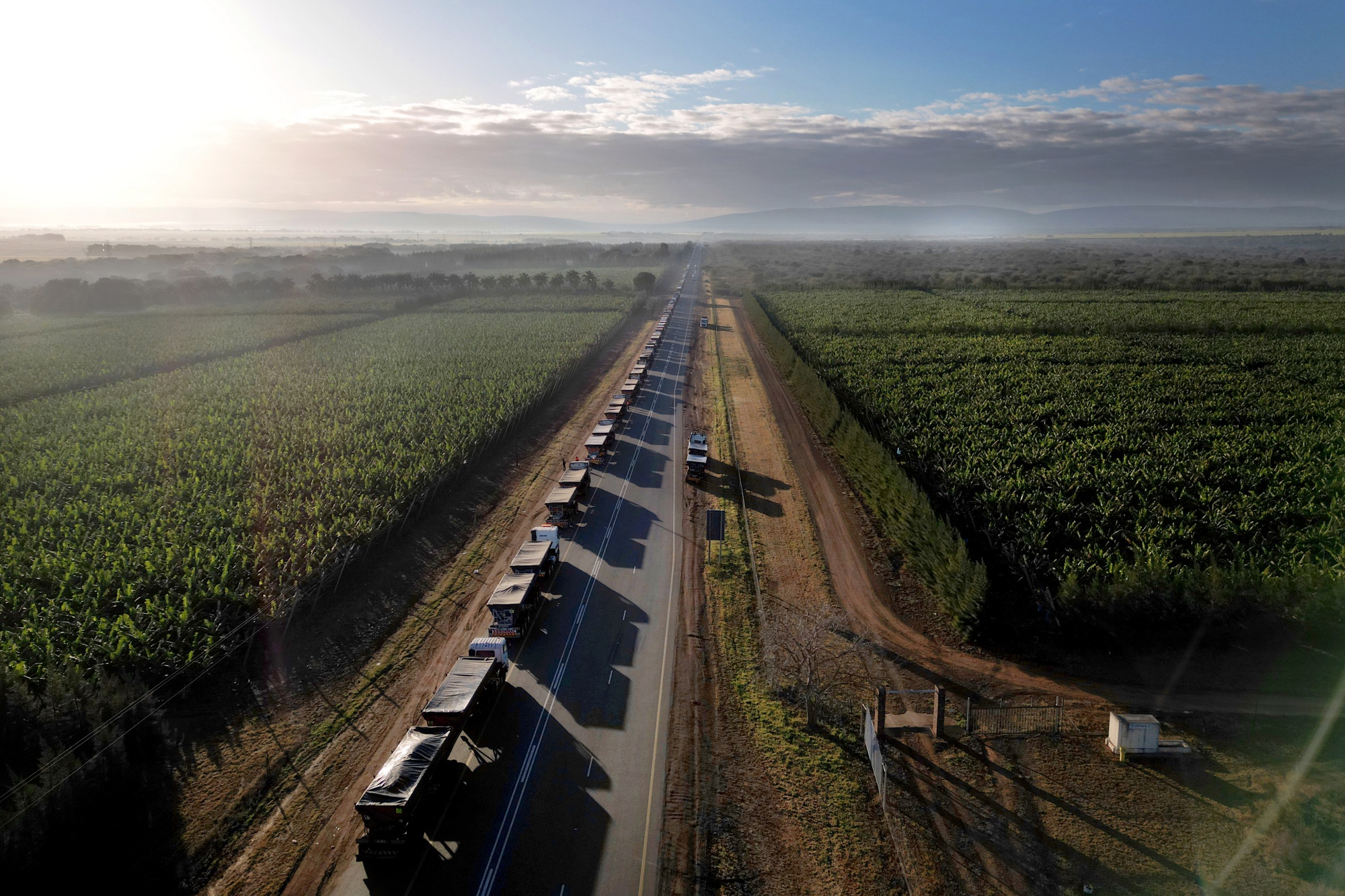The photograph captures an aerial view, likely taken with a drone, of a Midwest countryside road cutting through well-developed crop fields, possibly corn. The straight, two-lane roadway is lined with a convoy of over 10 trucks with tarps over their beds, stretching far into the distance and almost blending into the horizon. The bright green fields flank both sides of the road, neatly divided into rectangular sections. In the distance, the horizon is marked by a mix of pale blue sky and ominous rain clouds, with fog and slight hills visible. The top left corner of the image features a very bright area indicating the presence of the sun, casting long shadows across the road, suggesting that the photo was taken around high noon.